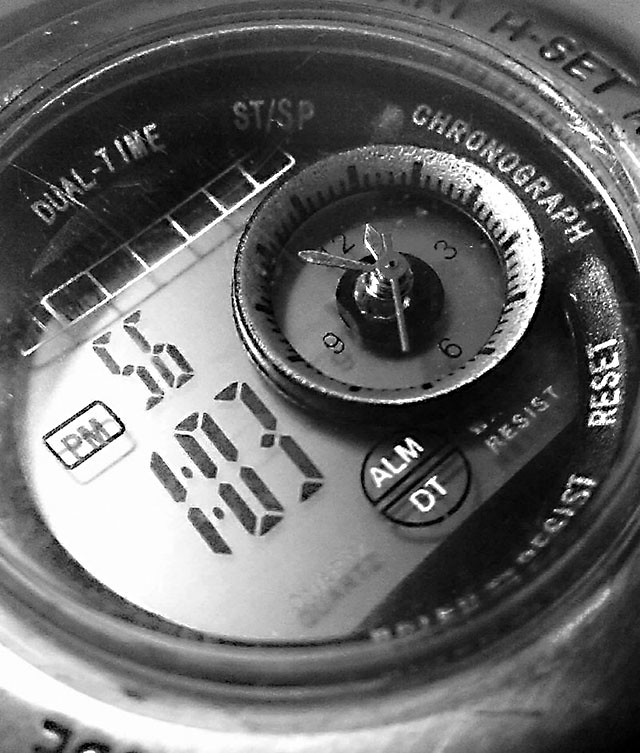This close-up black and white image showcases the intricate face of an elaborate watch, with the perspective so tight that the entire watch face isn't fully visible. The watch appears to have a robust outer casing made of either metal or hard plastic. On the side of the watch dial, the inscription "H-Set" can be discerned.

The interior of the watch is a fusion of digital and analog displays. The digital portion prominently displays the time "1:03 PM" in seven-segment format, along with the number "56". Surrounding this digital readout, the inside of the watch face features several labels, including "Dual Time", "ST/SP Chronograph", "Water Resist", and "Reset", all printed beneath the protective glass or plastic cover.

Central to the watch face, a smaller, sunken circular analog display resides, complete with minute, hour, and second hands. This analog section includes the numbers 3, 6, 9, and 12, providing a traditional timekeeping element amidst the modern digital interface. The hybrid design of this watch highlights a sophisticated blend of old and new technology, encapsulated within a carefully crafted, durable casing.